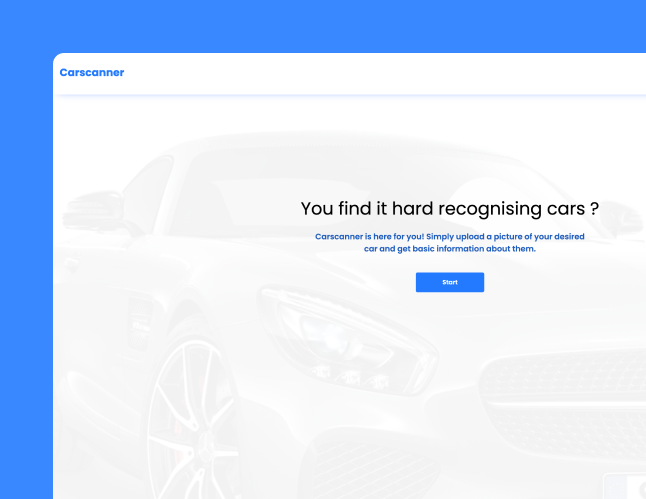This image showcases the main page of a website dedicated to identifying and providing information about cars. The webpage is designed within a rectangular frame, featuring a prominent bright blue background on the far left-hand side and the top of the page. Overlaid on this background is a central white box with a layout focused on user-friendly design.

In the top left corner of the white box, blue text reads "Car Scanner," establishing the website's brand. Dominating the middle of the page, bold black lettering poses the question, "You find it hard recognizing cars?" Beneath this, in smaller blue text, the instruction is provided: "Car Scanner is here for you. Simply upload a picture of your desired car and get basic information about them." This suggests that the website functions primarily as a tool for users to obtain essential details about any car by uploading an image.

While the specific use cases—whether for repairs, purchases, or general information—are not explicitly stated, the service's simplicity is emphasized. Below the descriptive text lies a small blue button labeled "Start" in white letters, inviting users to begin the process. The page appears to be introductory and user-friendly, likely offering guidance on the next steps upon clicking the "Start" button. The overall design is minimalistic, with the available information encouraging user interaction through the clearly defined start button.